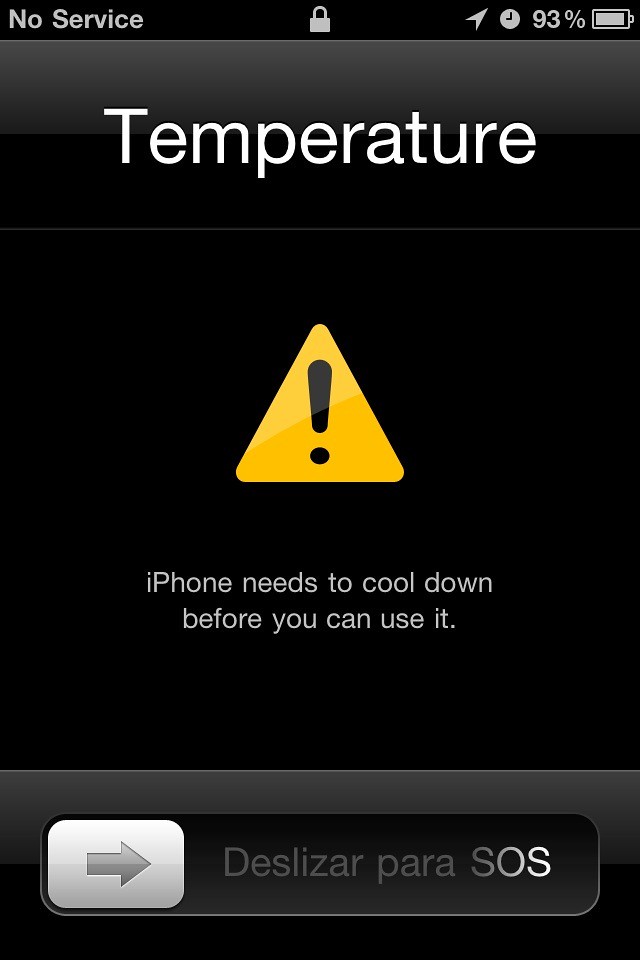This image is a vertically cropped screenshot of an iPhone screen displaying an overheat warning message. At the top-left corner, the status bar shows "No Service" in black text on a white background. In the center top, there's a small, locked padlock icon in white. On the top-right, there are several icons also in white: an upwards-pointing arrow, a clock symbol indicating an alarm or timer is set, and a battery icon showing 93% charge. Dominating the center of the screen is the word "Temperature" in white text against a black background. Below it, there's a yellow triangle warning symbol with a black exclamation point. The accompanying warning message states, "iPhone needs to cool down before you can use it," in white text. At the bottom of the screen, there's a black or light gray bar containing a rectangle with a white right-pointing arrow. To the right of this rectangle, in grey text that turns white near "SOS," it reads "Deslizar para SOS." This bar suggests a slide mechanism for emergency SOS activation.